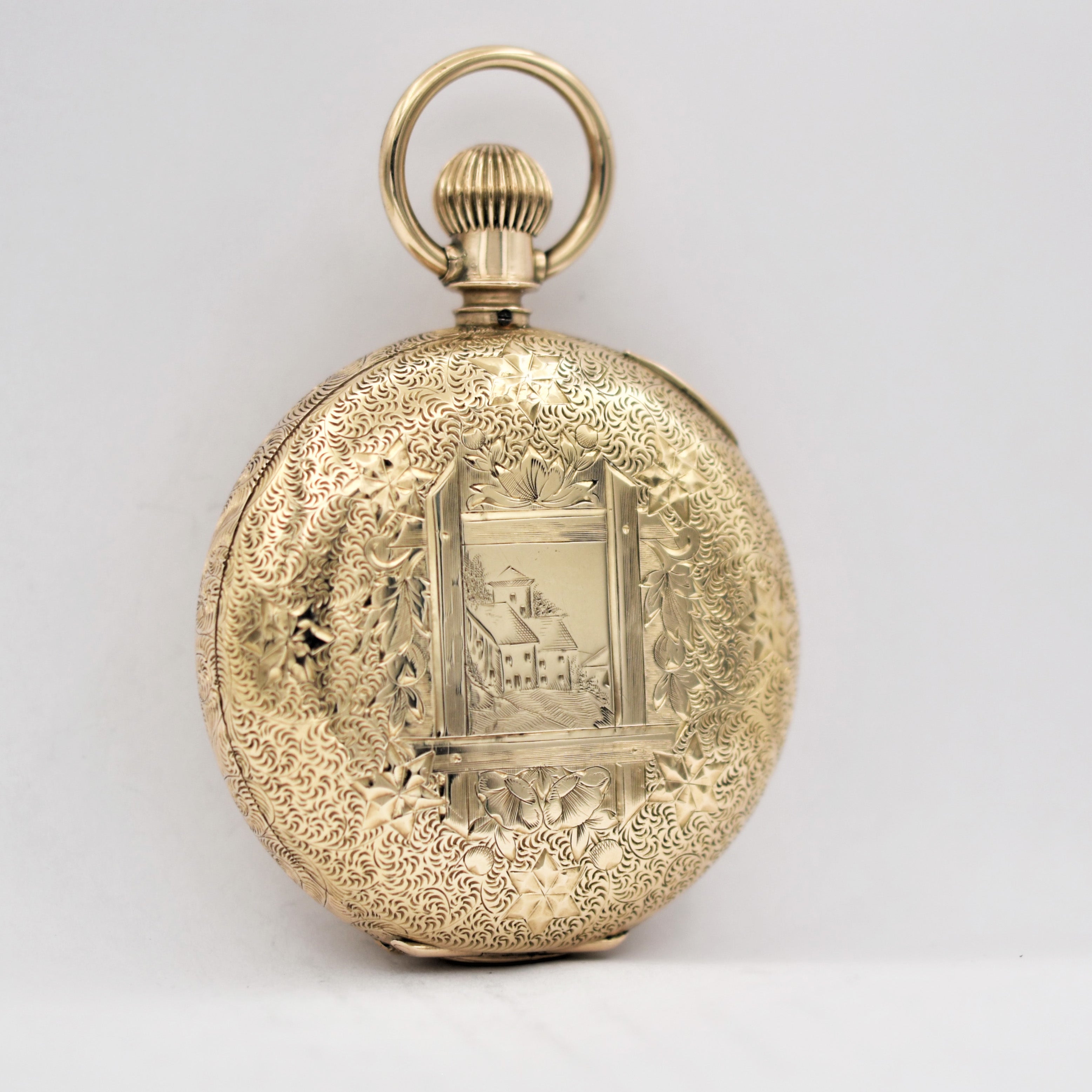This image captures an ornate, vintage pocket watch made of brass with a rich patina, giving it an aged appearance. The pocket watch is closed, showcasing a meticulously hammered metal case adorned with intricate floral and organic designs. At the very top, there is an actuator button accompanied by a ring, allowing it to be attached to a chain for carrying. The centerpiece of the design features a detailed, framed image of a countryside landscape, complete with several buildings, possibly farmhouses with windows and a lawn in front. Surrounding this central image is a spiral pattern, adding to the overall intricate craftsmanship. Notably, the design also includes an ornate depiction of branches or tree tops with small plants and a single gold butterfly near the bottom. The entire watch exhibits a high level of detail and craftsmanship, suggesting that it took a considerable amount of time and skill to create.